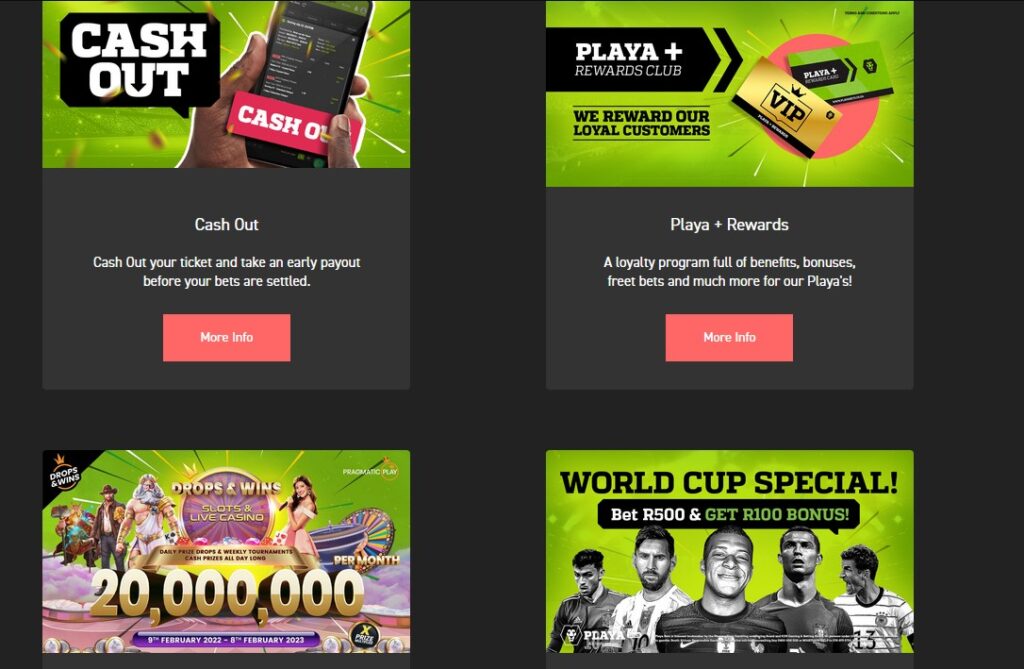The image is composed of four individual pictures arranged in a two-by-two grid against a grey background, creating a cohesive setup that implies their association.

1. **Top-Left**: The first image showcases the title "Cash Out" with a description encouraging users to cash out their ticket and take an early payout before their bets are settled. A "More Info" button is also visible for additional details.
   
2. **Top-Right**: The second image highlights the "Player Plus Rewards" program, which is a loyalty scheme offering a range of benefits, including bonuses and free bets for players. Notably, there is a typographical error where "free bets" is misspelled as "freet bets."

3. **Bottom-Left**: The third image, titled "Drops and Wins," features a vibrant scene with various characters designed to evoke the excitement of a jackpot or video game atmosphere. The caption promotes a substantial prize pool of 20 million (currency unspecified) and specifies the event duration from February 9, 2022, to February 8, 2023.

4. **Bottom-Right**: The final image advertises a "World Cup Special" offer where users can bet R500 and receive a bonus of R100, presumably in the same unspecified currency.

Each image contributes to a broader narrative of promotions and offers, targeting gamblers and players with diverse interests and incentives.